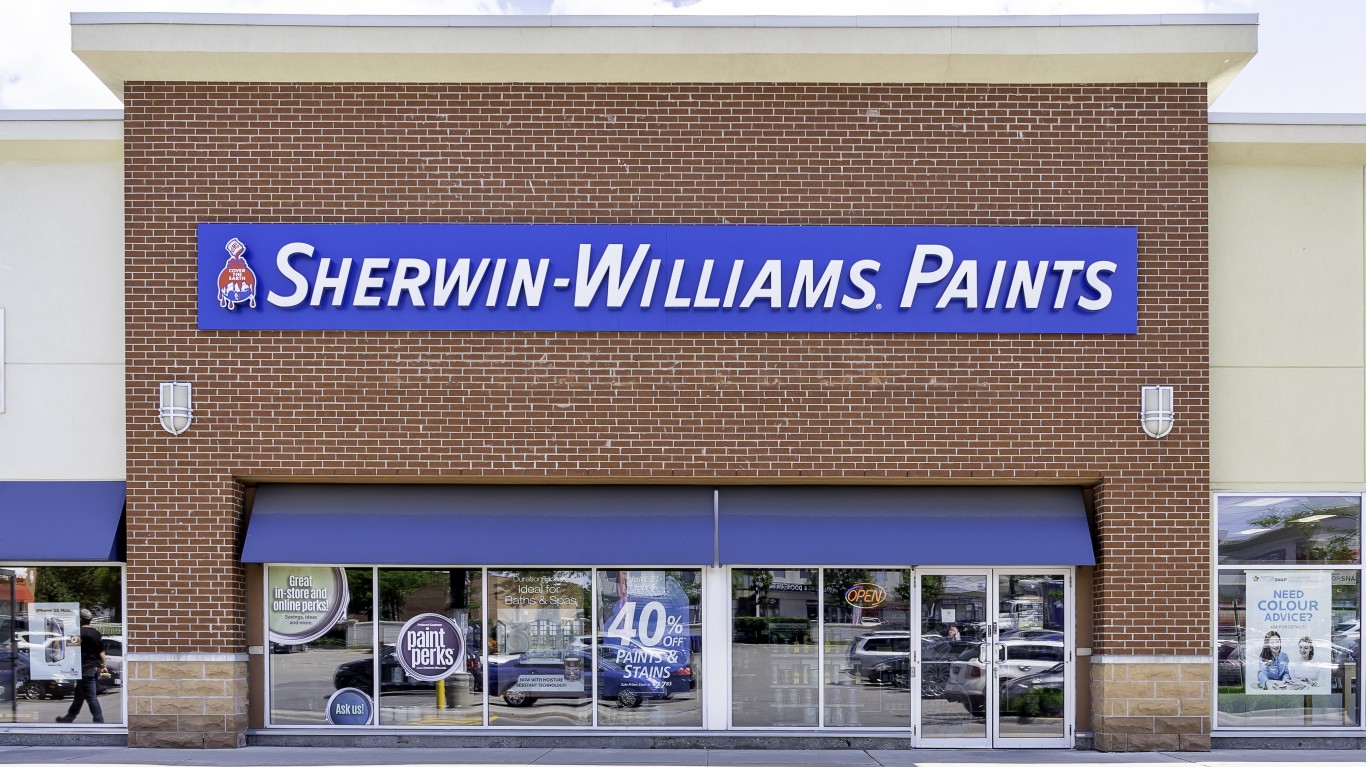The image captures an outdoor scene featuring a Sherwin-Williams Paints store, distinguished by its brick façade. Prominently displayed above the awning and doorway is a bold blue sign with the white text "Sherwin-Williams Paints," accompanied by the brand's iconic red, white, and blue logo. At the ground level, a sidewalk stretches in front of the store, which features two blue awnings that shade a long glass window and a pair of double glass doors to the right. The glass surfaces reflect the parking lot, revealing numerous cars and a strip mall building. Additionally, a white sign on the right side of the brick building's façade invites passersby with the message, "Need color advice?"